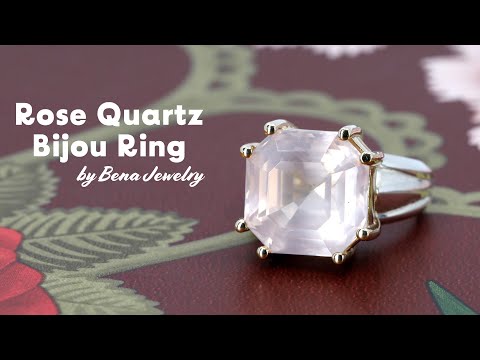The image is a close-up photograph of an octagonal-shaped ring, prominently featuring a faceted stone that appears clearish white, resembling quartz. The ring is set with eight prongs around the corners and is mounted on a silver band. It is positioned on a wooden table, adorned with a maroon floral design that includes drawn red petals, green leaves, and a stem. The photograph has black borders at the top and bottom, giving it an advertising feel. White bold text to the left reads, "Rose Quartz Bijou Ring by Benna Jewelry," highlighting the product and its maker.